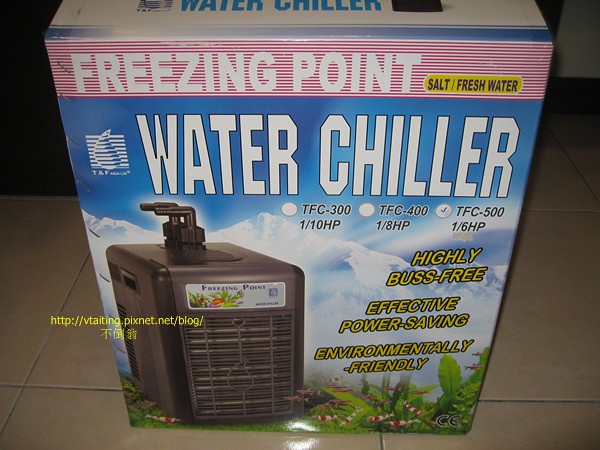The image shows a product packaging for a water chiller. The top features a red and white striped lining with the brand name "Freezing Point" prominently displayed. Next to the brand name, there is a small yellow box that states the chiller's compatibility with both "salt/fresh water." Below it, the Alpine background boasts snowy mountains and blue skies, contrasting with the green vegetation in the foreground where the product is showcased. 

The water chiller itself is a sleek black box, equipped with black vents and two black pipings on top. Right above the product image, large white text reads "Water Chiller." Next to the product are three model specifications: TFC-301-10HP, TFC-401-8HP, and TFC-501-6HP, with a checkmark beside the TFC-501-6HP model, indicating it's the featured version. Additionally, the packaging highlights key features of the chiller in yellow text: "Highly bus-free, effective power saving, and environmentally friendly."

The visual and textual elements together emphasize a high-performance water chiller designed for efficiency and eco-friendliness.